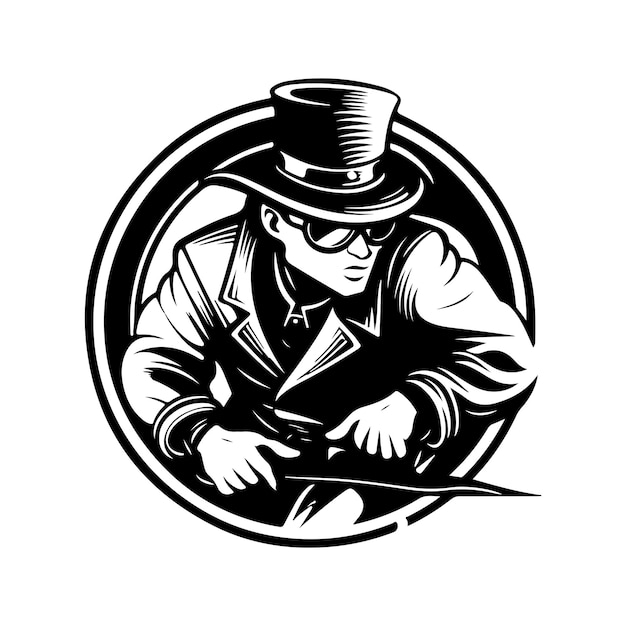The image is a black-and-white, hand-drawn illustration with a circular composition. At the center of the image is a somewhat nefarious character, possibly inspired by comic books or steampunk aesthetics. The man, depicted from the torso up, wears a top hat with a ring around it and dark sunglasses that conceal his eyes. His facial features include a sharp, pointy chin and nose, and he has a stern, serious expression. He dons a trench coat with a visible tie or necklace underneath. In his right hand, he holds a short dagger or knife, poised as if ready to lunge out of the frame. The drawing lacks a background, focusing entirely on the character who is set against a deliberately used white space. Surrounding him are alternating black and white rings that form a thick circular border enclosing the image.